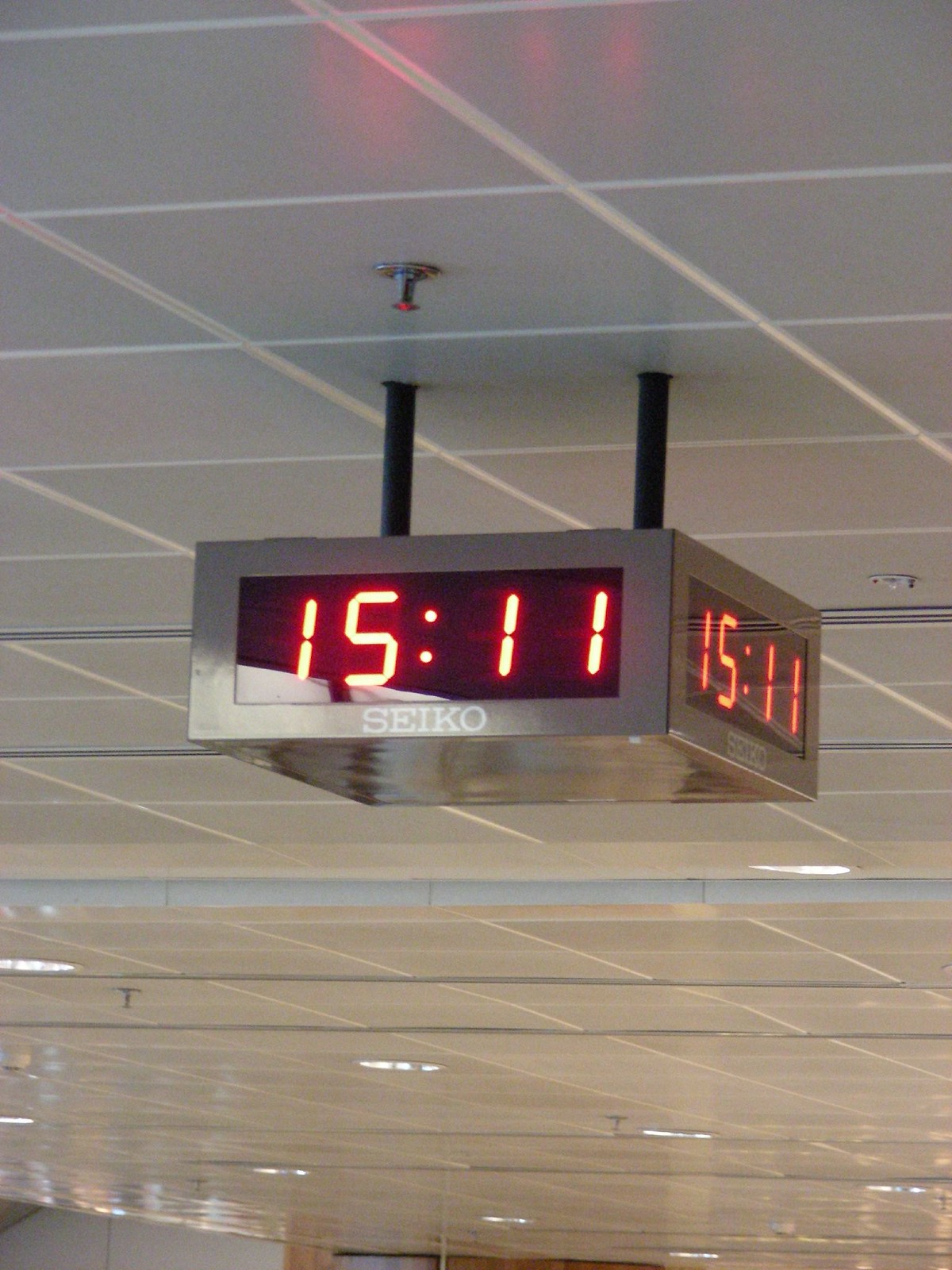The image showcases a large, rectangular digital clock suspended from a dark gray, tiled ceiling by two black poles. The clock, which displays the time in military format as "15:11" in vibrant red digits, is produced by the brand Seiko, with its name written in white on the clock. The clock's body is made of stainless steel, and the digits contrast against a black background for easy visibility. The clock has displays on all four sides, but only two sides are visible in this perspective. The ceiling features numerous light fixtures arranged in a circular pattern, adding a reflective sheen to the ceiling tiles, while reflections of the red digits can also be seen in these tiles. Some ceiling tiles appear white or beige in the gaps between the dark gray sections, and there are additional details like sprinklers visible against the varied colors of the ceiling tiles.